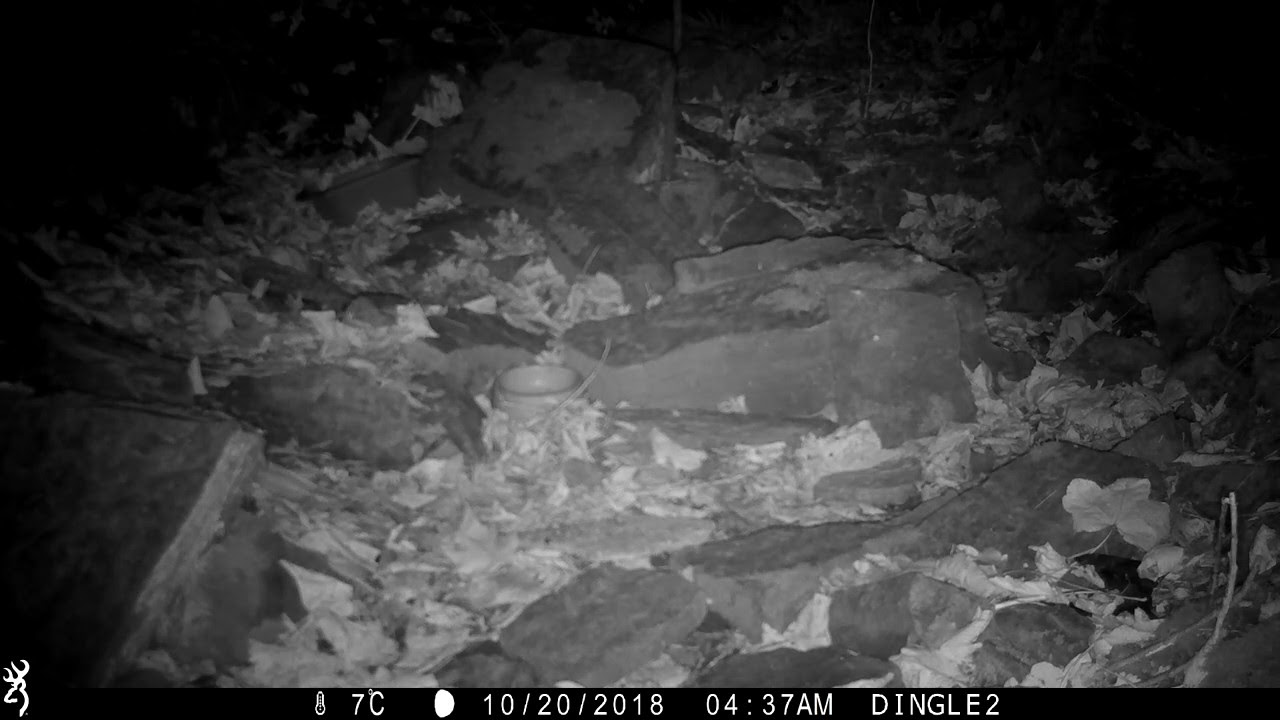This black and white security camera image, taken outdoors at night and timestamped 10-20-2018 at 4:37 a.m., captures a natural setting in low light. Central to the composition is a small bowl or cup positioned near some rocks. Scattered around these rocks are numerous leaves and sticks, creating a rugged, natural atmosphere. In the background, there appear to be trees, adding to the scene's outdoor ambiance. The temperature at the time of the snapshot was 7 degrees Celsius. The image, devoid of visible animals, features a bottom rectangular overlay in white text detailing the date, time, temperature, and a label "Dingle 2." A small gear icon or logo is also present. Despite the darkness making certain elements indistinguishable, the composition distinctly reflects an early morning, pre-dawn moment captured by a trail cam.